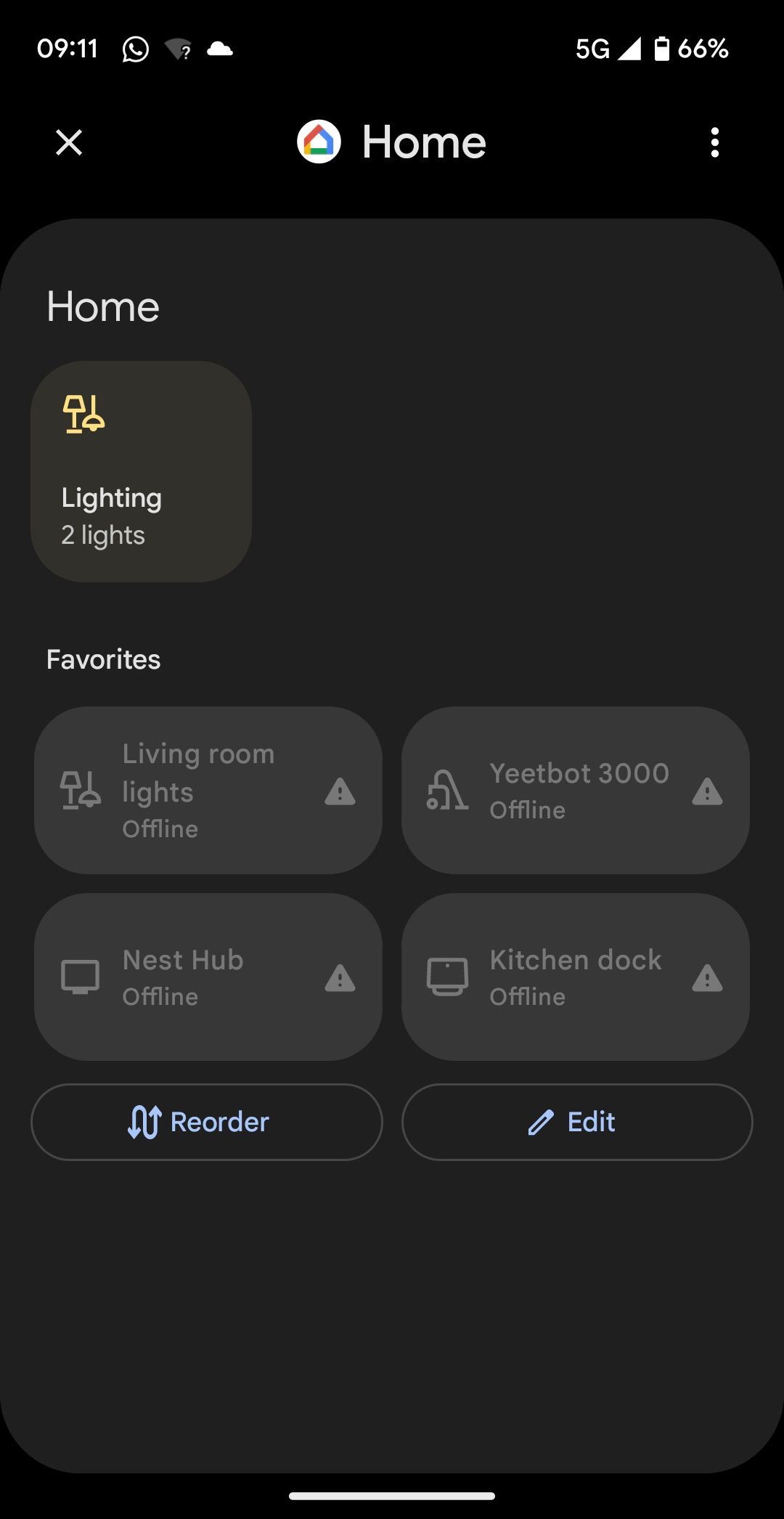Screenshot of a Mobile Google Home Page with Dark Theme:

The screenshot features the Google Home app in dark mode. The background is primarily black, with varying shades of black for different informational sections. 

**Status Bar (Top Right Corner):**
- Time displayed in white: "09:11"
- Quotation bubble with a phone icon inside.
- Grayed out Wi-Fi icon resembling a pie shape with a white question mark, indicating unknown signal strength.
- Cloud icon next to the Wi-Fi indicator.
- "5G" text indicating network type in the upper right corner.
- Right triangle with an adjacent right-angle corner, situated in the bottom right of the status bar.
- Vertical battery icon displaying "66%".
- White X icon next to the battery level.

**Main Page:**
- Google Home logo embedded in a white circle, accompanied by the word "Home" in white text and three vertical dots for the menu.
- The main section header in white text: "Home".
- A sizable box with rounded corners, a yellowish-black background, and an icon representing a combination of a floor lamp and a ceiling lamp, suggesting lighting controls.

**Favorites Section:**
- Labelled "Favorites" in white text.
- Features a 2x2 grid layout:
  - Top Left: Living Room Lights (offline, indicated by a greyed-out warning triangle).
  - Top Right: YeetBot 300 (offline, indicated by a greyed-out warning triangle).
  - Bottom Left: Nest Hub (offline, indicated by a greyed-out warning triangle).
  - Bottom Right: Kitchen Dock (offline, indicated by a greyed-out warning triangle).

**Action Buttons:**
- Reorder button with a black background and grey outline, marked by an S-shaped arrow with arrowheads facing up and down.
- Edit button featuring a greyish-blue pencil icon and text "edits" against a black background with a grey outline.

**Footer:**
- Centralized white rectangular bar, approximately 30% of the screen's width.